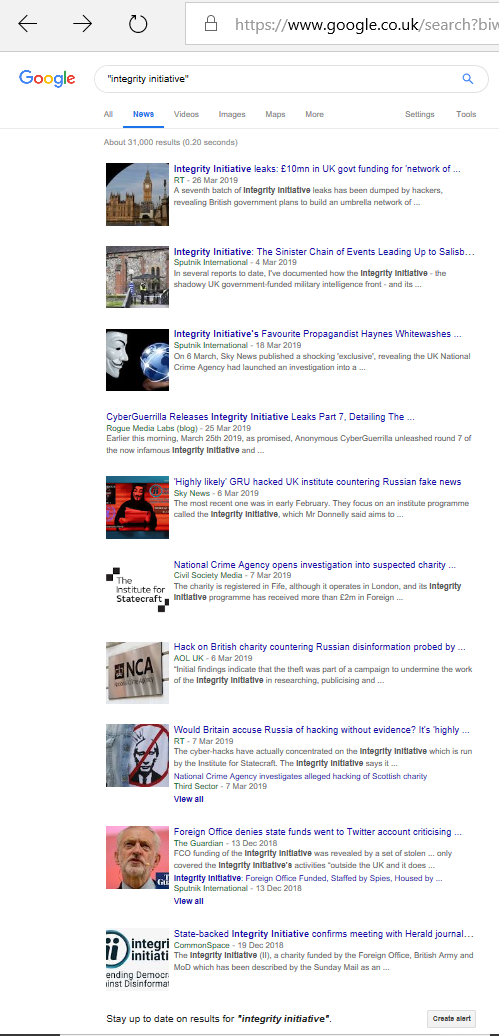Screenshot of a Google search on google.co.uk for "Integrity Initiative," displaying results under the "News" tab. The search results show approximately eight to nine articles. Each result features a thumbnail image on the left, followed by the article headline. The first headline reads "Integrity Initiative Leaks," while the second mentions "Integrity Initiative: The sinister chain of events leading to..." and is truncated with an ellipsis. The Google search interface is partially visible, missing the top navigation bar and not showing the bottom of the page. Typical Google search formatting is present, with headlines in blue and brief summaries in gray text below. There is no visible date or time stamp on the screenshot.